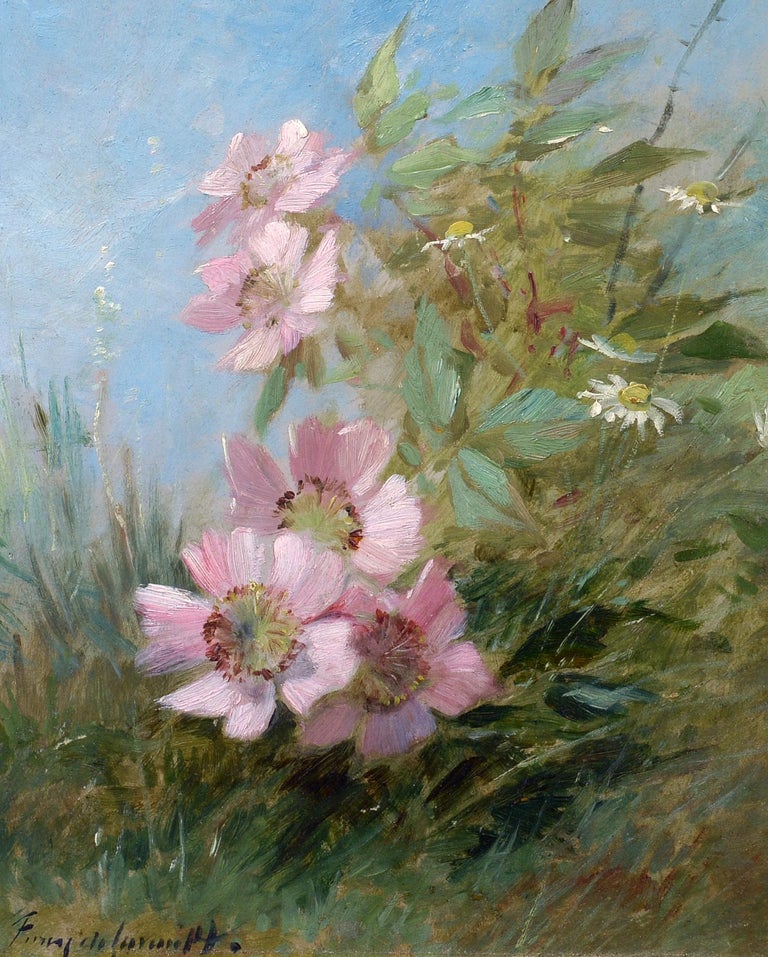This is a detailed painting, possibly an oil or acrylic piece with an impressionistic style reminiscent of older French painters. It depicts an outdoor scene featuring a bunch of light pink flowers with delicate, almost whimsical petals and vibrant centers that transition from red to yellow. The painting’s texture is loose and flowy, capturing movement with brushstrokes that convey the flowers and grass swaying in the wind. 

At the forefront, situated more towards the left, are three prominent flowers with intricately detailed centers resembling dandelion puffballs. Above, two more flowers peak through against a sky that fades from blue to light gray, evoking an early spring morning. Interspersed throughout the scene is greenery, with a blend of deep and pale greens, some almost discolored to orangey hues, providing depth and contrast. Whisps of pale green leaves and grass add to the impressionistic, dreamy quality of the painting.

On the right, more greenery frames the composition alongside white flowers with striking yellow centers. Overall, the painting blends detailed and broad brushstrokes to create a sense of depth, making the flowers in the foreground appear closer. The artist’s signature is located at the bottom left in black paint strokes, though it is not legible.